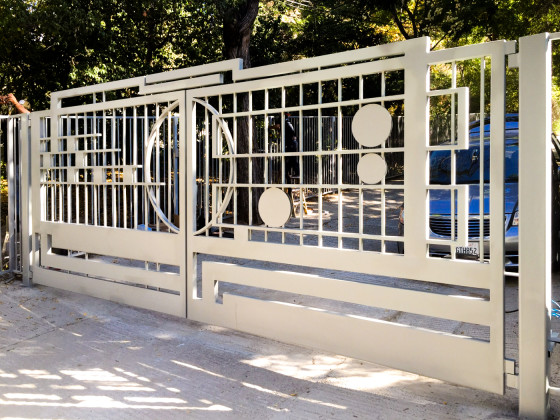This is a color photograph of a large, white metal gate adorned with various ornamentations, including circles, rectangles, and squares. The gate is designed to open in the middle, and it stands on a concrete driveway. Behind the closed gate, you can see a car, possibly a Mercedes, partially obscured by the metal grid. Beyond the car, the background reveals a tree-lined, wooded road, adding to the serene outdoor setting. Additionally, there appears to be a man standing to the left of the gate, contributing to the scene's sense of place and scale.